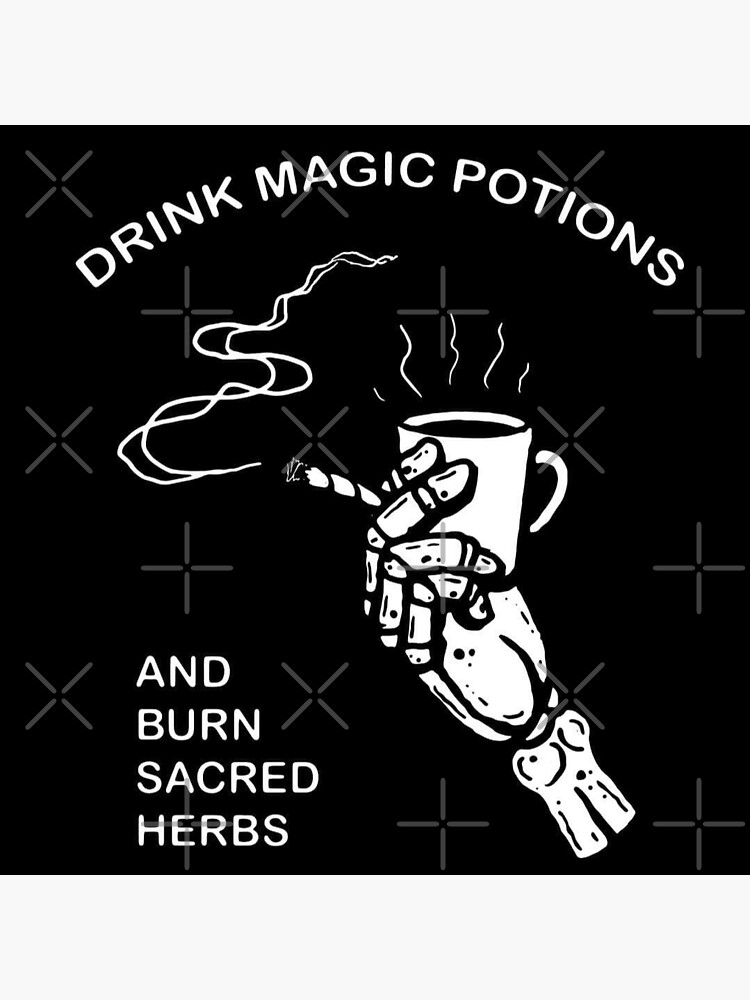This is a black-and-white poster with a black background featuring scattered translucent plus and X shapes. At the center, a white skeleton hand is depicted holding a steaming cup of coffee and a lit cigarette emitting squiggly smoke lines. In a crescent, rounded design at the top, white text reads "DRINK MAGIC POTIONS," while in the lower left corner, more white text states "AND BURN SACRED HERBS." The detailed design suggests an advertisement or artwork that could also appear on a shirt.